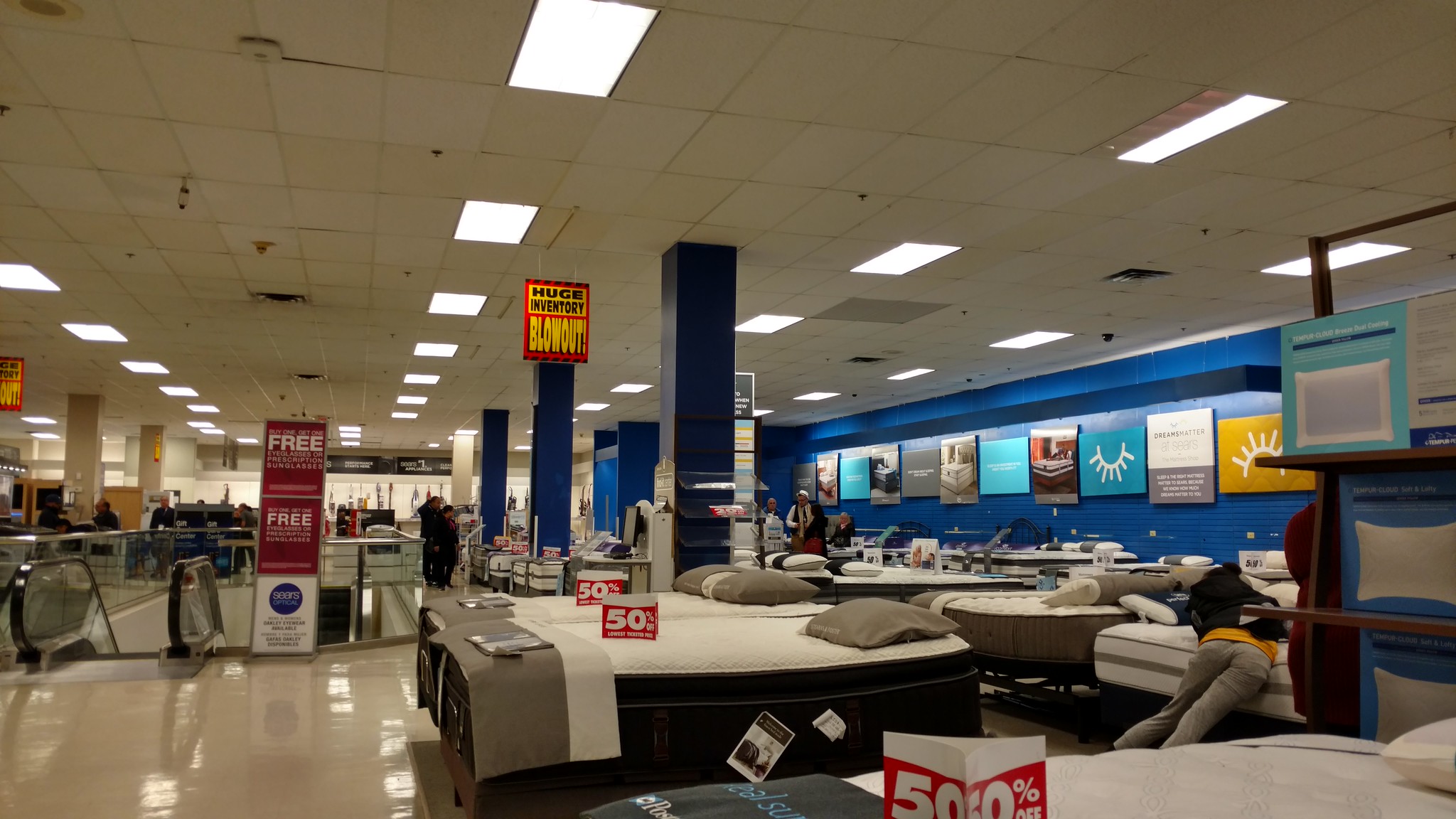The image depicts the mattress section of a bustling department store, showcasing a wide array of products. Prominent signs indicate a massive 50% off sale as part of a huge inventory blowout, with one such sign affixed to a pillar. The section's walls are painted a calming blue, and numerous beds are neatly arranged across the floor. 

A visually striking aspect is a person wearing gray pants, an orange shirt, and a black jacket, who appears to be leaning half on, half off a mattress, perhaps testing its comfort. Along the blue wall, various advertisements for different mattress types are visible, some featuring cheerful smiles with lines extending downward, and one illustration that resembles a radiant sunshine.

Notably, escalators facilitate movement within the store, descending to other levels. A red sign in the background announces a "free" offer, though the details are not legible in the image. The expansive store floor is filled with merchandise extending into the distance, with other shoppers browsing through the selections, contributing to the vibrant and busy atmosphere.